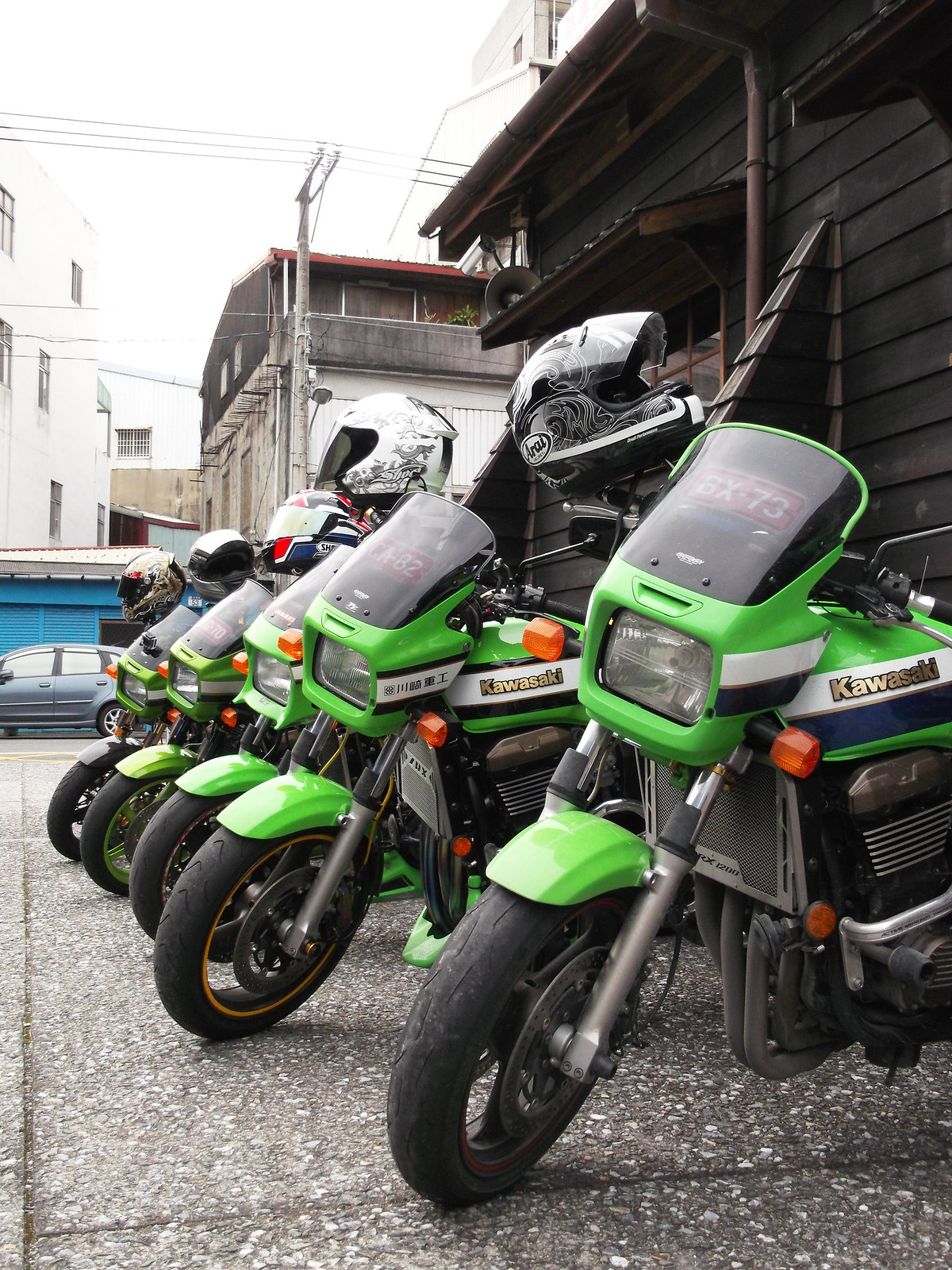This is an outdoor photograph taken within a city next to some older wooden buildings. The vertically aligned rectangular image captures a row of six green Kawasaki motorcycles lined up along a sidewalk composed of large, speckled gray and white square sections. Each motorcycle is adorned with a helmet hanging from the right handlebar, featuring various colors and designs, including black, white, red, blue, and brown with ornate patterns. Prominently, "Kawasaki" is written in gold on the left side of each bike. The motorcycles, possibly dirt bikes due to their appearance, are neatly parked, showing only the front tire and the left side of the first two bikes clearly, while the rest fade into the background. The front of each motorcycle has orange lights, black tires, and a large, square-shaped window. In the distant background, additional buildings, a car, a blue garage, and power lines are visible under a bright, white sky at the top left corner of the image.